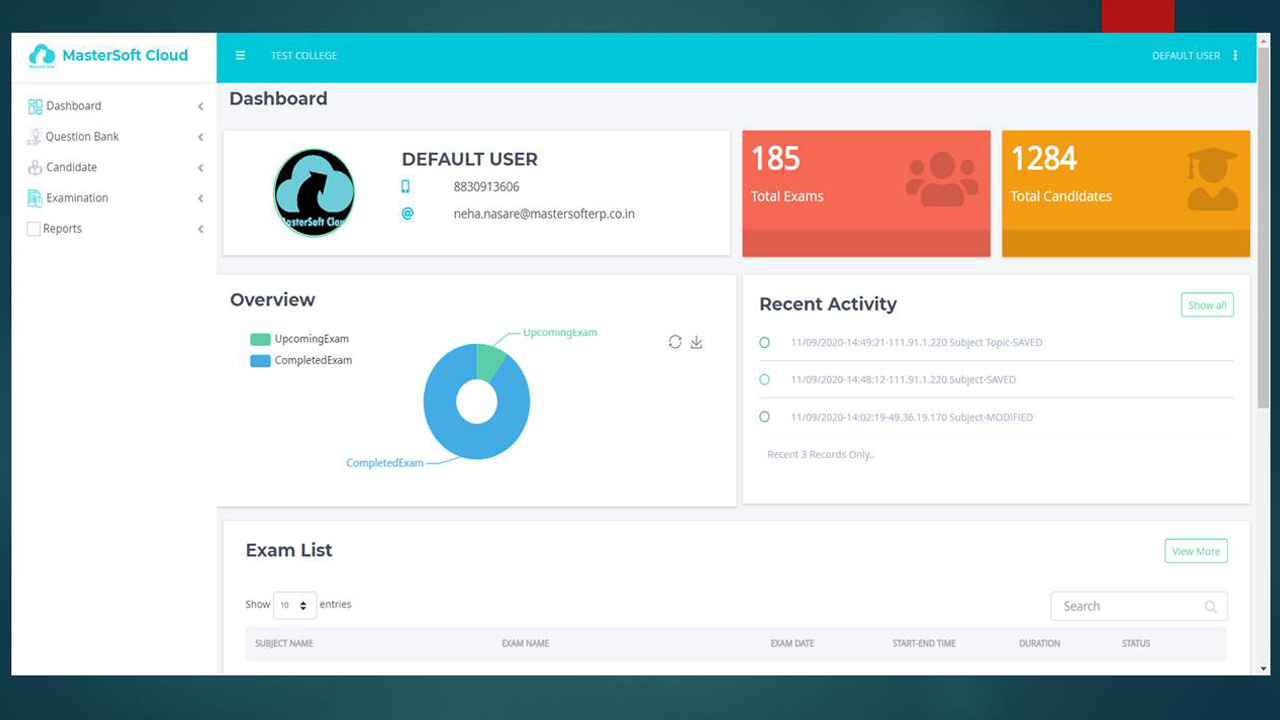This image depicts a detailed view of a website interface, featuring multiple sections with varying functionalities:

- **Header Section**: The very top of the interface features a thin black bar across the width of the screen. Towards the right end of this bar is a small red section. 

- **Branding and Navigation Bar**: Beneath the black bar is a broader, blue bar with a gradient transitioning to white on the left. On the left side of this bar, the text "Master Soft Cloud" is displayed in a teal hue, accompanied by a cloud logo. There are three vertical white lines symbolizing a menu. Beside these lines, the words "TEST COLLEGE" appear in all caps. On the right side of this blue bar, the text "Default User" is displayed next to a vertical stack of three dots.

- **Sidebar**: On the left side of the screen, spanning from the top to the bottom, is a vertical menu bar. The sidebar's background is white and contains the following menu items: "Dashboard", "Question Bank", "Candidate", "Examination", and "Report", each paired with an icon and left-facing arrows.

- **Main Content Area**: 
  - Below the blue branding and navigation bar, on the left, "Dashboard" is written with white space to its right.
  - In the middle of the screen is a prominent white box displaying a cloud logo with an arrow through it. It includes "Default User", a phone icon followed by the number "8830913606", and an email address "NIHA.NASERI@mastersofterp.co.in". 
  - Two colored boxes are positioned under this: a red box with the text "185 total exams" in white, and a yellow (golden) box with "1284 total candidates" in white.
 
- **Analytics Section**: Within the same area to the left, a white box is labeled "Overview". Inside, it displays "Green: Upcoming Exam" and "Blue: Completed Exam". A pie chart is centered within this box, mostly filled with blue signifying completed exams, with a small green wedge indicating the upcoming exams.

- **Activity Log**: To the right of the analytics section is another white box titled "Recent Activity". It lists dated entries, all marked "11-09-2020", labeled as "Subject Topic Saved", "Subject Saved", and "Subject Modified". It is noted that these are the "Recent Three Records Only".

- **Exam List**: Beneath the "Recent Activity" box is the beginning of another section labeled "Exam List". This includes a header specifying columns such as "Subject Name", "Exam Name", "Exam Date", "Start Time", "Duration", and "Status". A search bar is positioned above these columns, although the detailed exam entries are not visible in this image.

The overall layout also includes black bars running vertically down each side of the interface and a thicker black bar along the bottom of the screen.